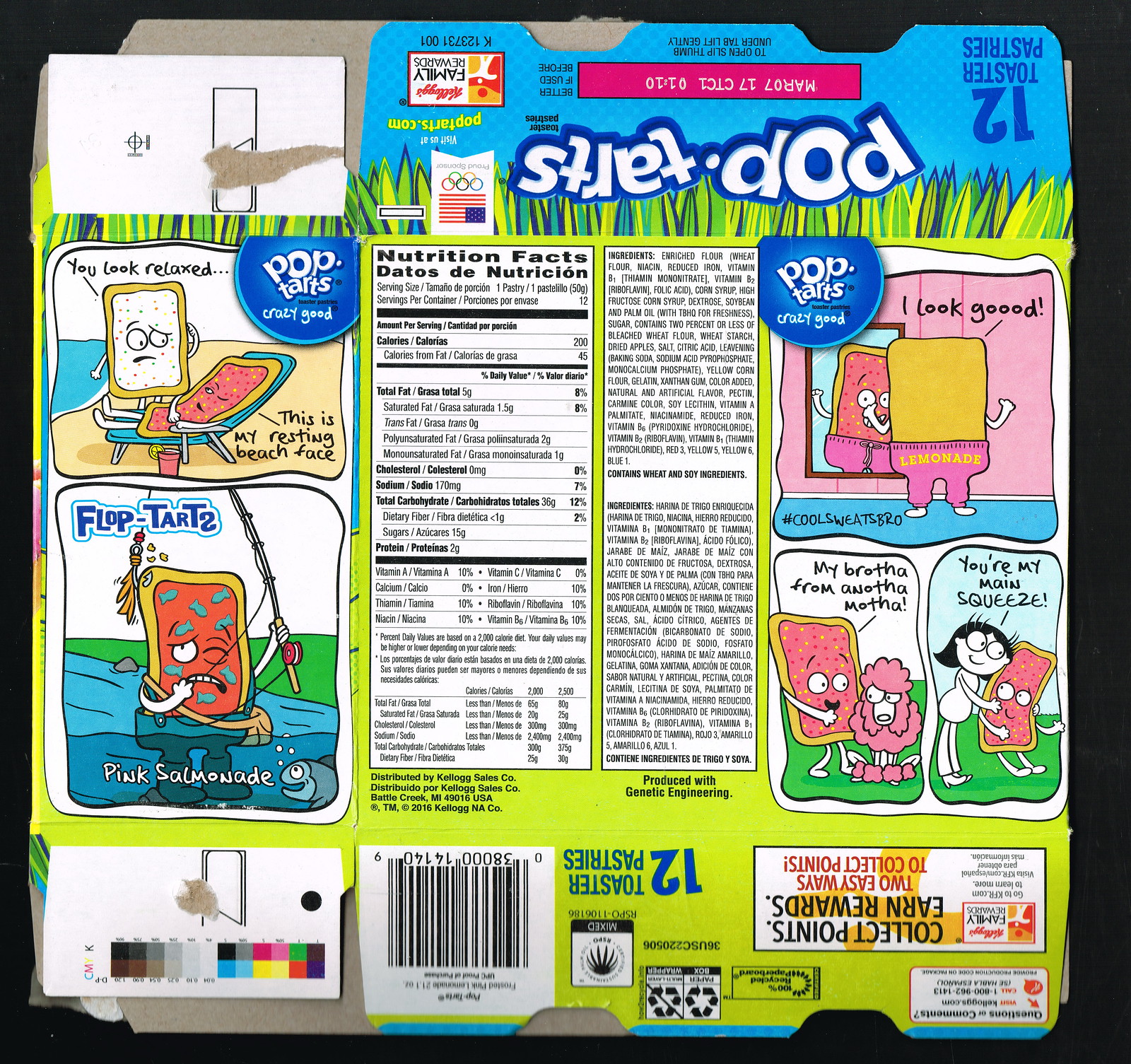This photo features a thoroughly deconstructed Pop-Tart box, meticulously laid flat to display all its surfaces. The image captures the back side, one of the side panels, the top flap, and the bottom of the box. The top flap, which is folded over and hence appears with upside-down text, indicates that the box originally contained 12 pastries and prominently displays an expiration date printed in pink. The phrase "Pop-Tarts" is emblazoned in a white font with a dark blue border, against a primarily green and blue background.

The center panel of the box showcases the nutrition facts, flanked by whimsical, comic-like illustrations of animated Pop-Tarts. One Pop-Tart character is lounging on a beach chair, another is indulging in fishing, a third is admiring itself in a mirror, and a fourth pair is depicted in an embrace. The bottom of the box includes a visible barcode. Overall, the photo is densely packed with details, creating an eclectic and detailed visual narrative of this popular food product's packaging.